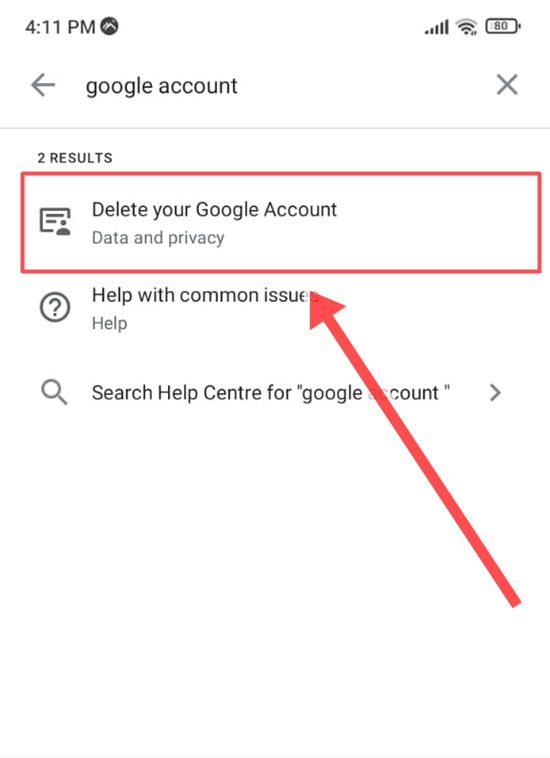This screenshot, captured on a mobile device at 4:11 PM, showcases a white background with dark gray text. On the top left of the screen, the time is displayed, while the top right shows icons for signal strength, Wi-Fi strength, and battery life, the latter being at 80%. Below, there is a user interface consisting of a text box flanked by a back icon (a left-pointing arrow) on the left and a clear icon (an 'X') on the right. The text within the box reads "Google account."

The search results obtained for "Google account" display two options. The first result is highlighted with a thick red-bordered box and a prominent red arrow pointing to it, drawing attention. The options are organized with simple white and gray infographics and are titled "Delete your Google account" under which is the subtitle "Data and privacy," followed by the text "Help with common issues." The text beneath reads "Help," and there are more clickable links below. Additionally, a magnifying glass icon is visible, followed by the words "Search help center for 'Google account'," indicating it will navigate to a broader web search rather than an in-app query.